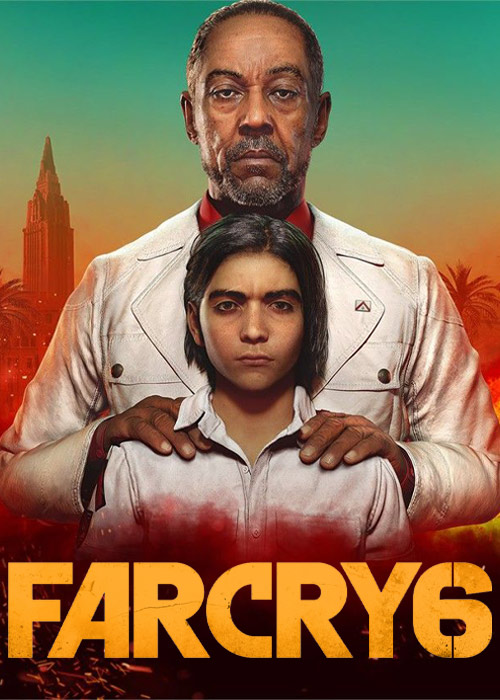The cover of the video game "Far Cry 6" prominently features the bold yellow title text at the bottom. Central to the image are two figures—a man and a boy—both facing forward with serious expressions. The man, an older black gentleman with short hair and a graying beard, stands behind the boy, resting his hands on the boy's shoulders. He is dressed in a white button-down coat over a red collared shirt. The boy in front, with shoulder-length black hair and bushy eyebrows, also wears a white collared shirt, with red hues creeping up the fabric. Their intense gazes are directed straight at the viewer. The background is a blend of green, yellow, orange, and red, suffused with red haze. To the left, a large skyscraper looms, and to the right, the silhouette of a palm tree adds to the vibrant and foreboding atmosphere.